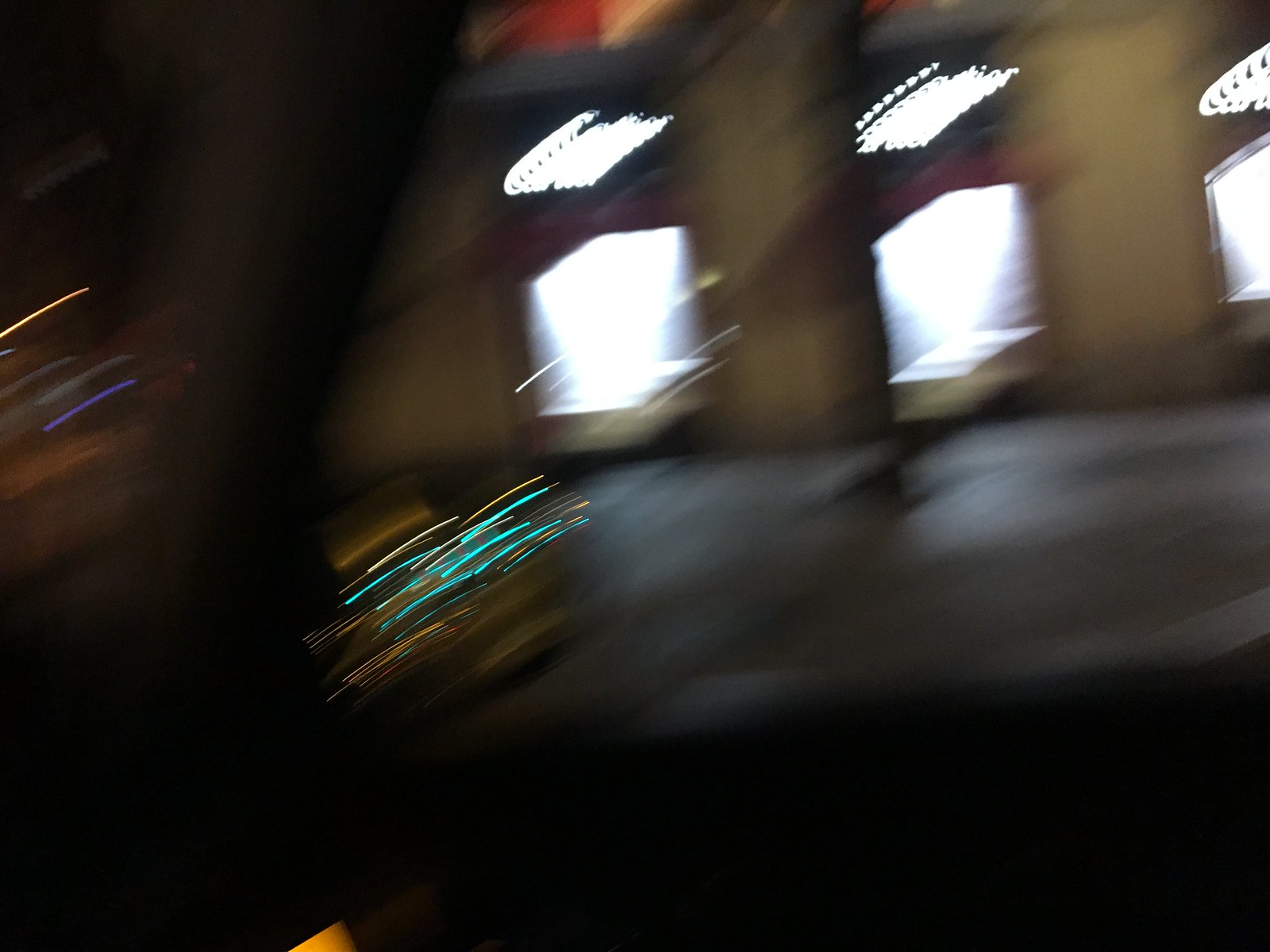The image is an extremely blurry, out-of-focus photograph likely taken from the inside of a moving car, as suggested by hints of a car door and potentially a rearview mirror in the shot. It captures a nighttime scene characterized by a building with multiple identical doorways or archways, illuminated by white light pouring out. Above these doorways are red and white stripes, while the ground in front of the building reflects the light, contrasting with the very dark foreground. Additional details include varied light sources: blue and white lights are positioned somewhat center-left, and purple and orange lights appear on the far left side. The dark sky and light streaks across the lens further reinforce the nighttime setting.